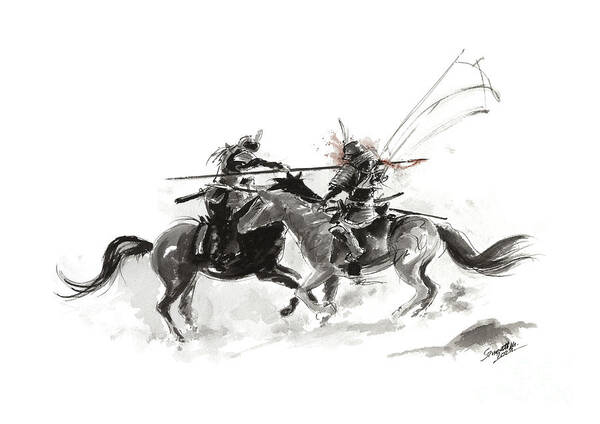The artwork is a detailed black and white sketch, likely done in charcoal, depicting an intense duel between two knights on horseback. Centrally positioned, the knights are engaged in a high-stakes joust. The knight on the left, mounted on a predominantly black horse with some gray shading on its hindquarters, has successfully speared the other knight. The deadly spear visibly juts through the victim’s back. The knight on the right rides a lighter, gray horse with a black tail. Despite the monochromatic palette, a subtle red tint suggests blood seeping from the shoulder wound of the impaled knight, adding a dramatic touch to the image. Intricate details include scattered lines and a signature at the bottom, hinting at the artist's identity. The drawing captures the dynamic motion of the duel, with hints of dust or plumes kicked up by the horses, emphasizing the chaos and intensity of the moment.